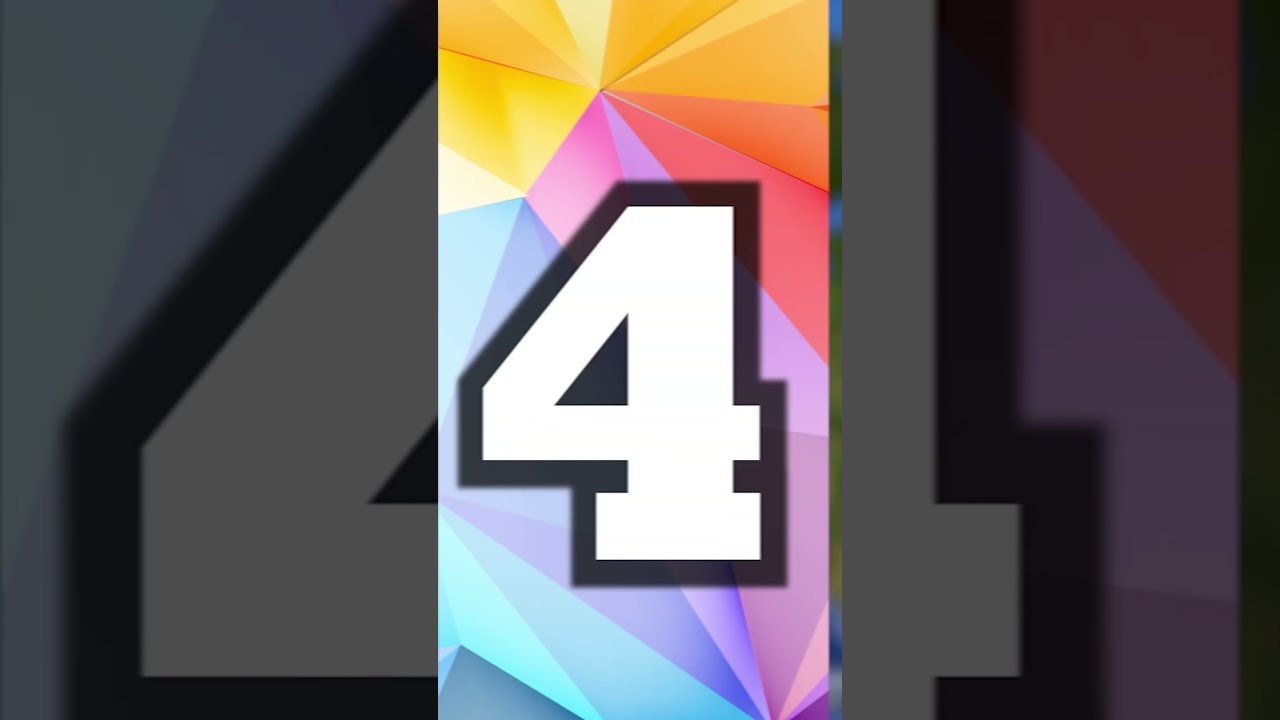This image is a wide, rectangular composite featuring a central vertical panel and darker, shaded close-ups on either side of the same panel. In the center, there's a tall, rectangular screenshot with a vibrant, rainbow-colored background that consists of triangular shapes fanning outward. The colors transition seamlessly from yellow at the top to orange, red, purple, pink, turquoise green, and finally to blue and green at the bottom.

Prominently displayed in the middle of this colorful backdrop is a large numeral 4, white with a black outline. The central panel has a distinctive design resembling folded origami paper, contributing to a layered, textured appearance. Surrounding this central image are side panels that are essentially close-up, darkened versions of the middle screenshot, adding depth and emphasizing the colorful, intricate details of the central design. The overall composition suggests a dynamic interplay of color and shape, with no additional text or indicators to explain the context or significance of the numeral 4.